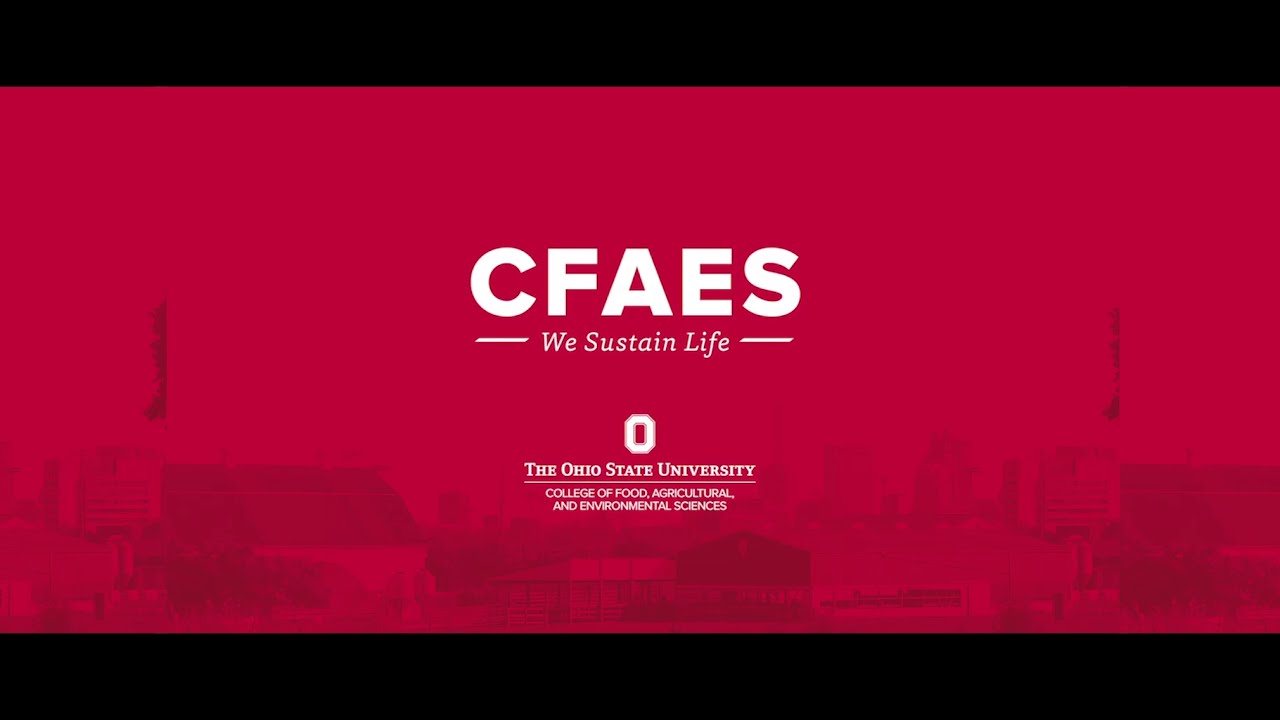This digital poster features a prominent central text that reads: "CFAES We sustain life Zero, The Ohio State University College of Food, Agricultural, and Environmental Sciences." The letters "CFAES" are in large, bold white fonts, while the remaining text is smaller and also in white. The background of the image displays a tinted scene of the Ohio State University campus, split with downtown buildings on the right and what appears to be agricultural or industrial buildings on the left. The entire image has a red overlay which dims and unifies the campus scene. The poster is framed by two horizontal black strips at the top and bottom. The detailed layout and prominent text suggest that this image might serve as a cover for a website or PowerPoint presentation related to the university's College of Food, Agricultural, and Environmental Sciences.